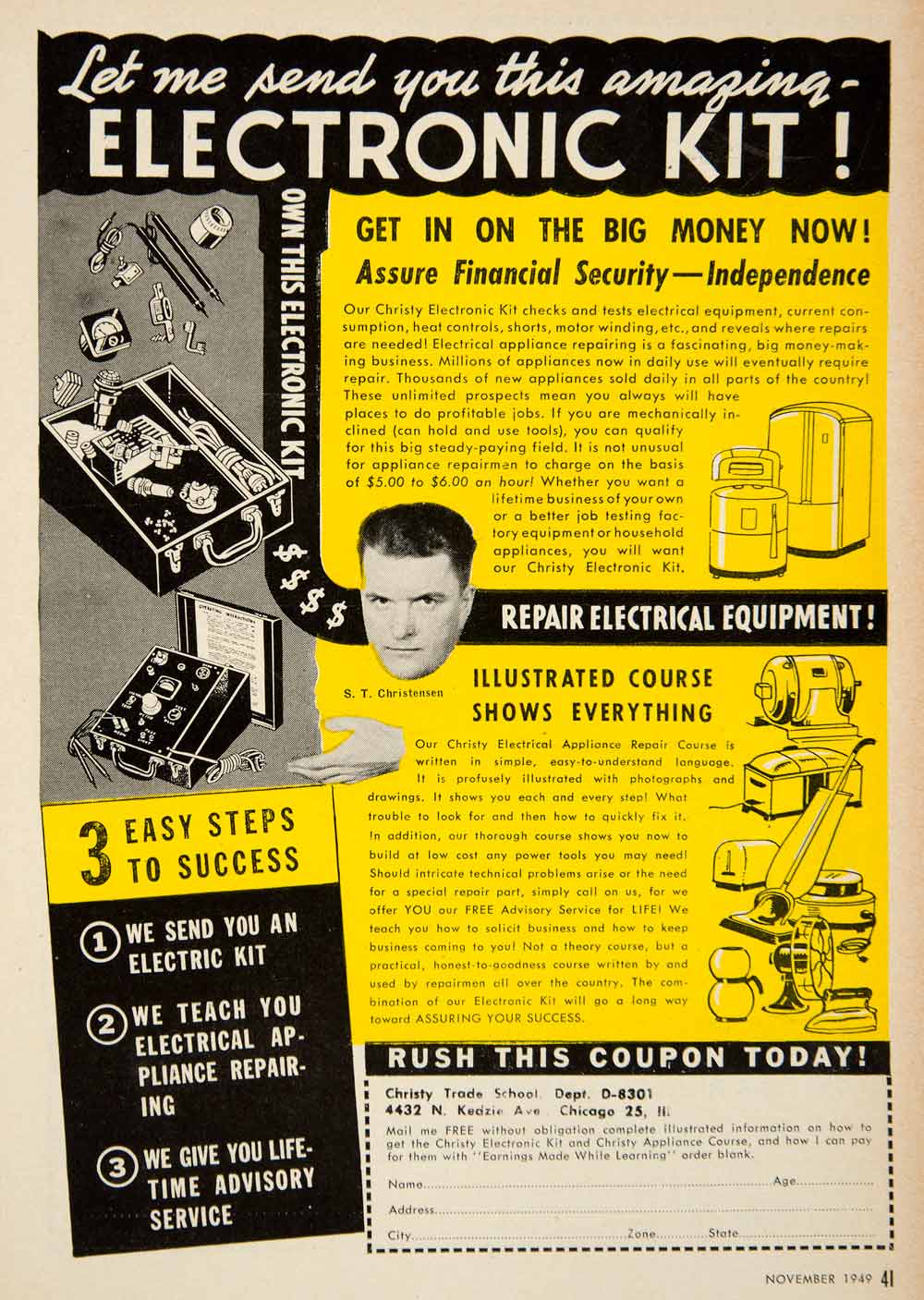The image is a vintage advertisement predominantly in yellow, black, gray, and white, enticing viewers to send away for an electronic kit. At the center of the image is a man's head, with his hand gesturing towards the "Three Easy Steps to Success." The steps indicate that the company will send the kit, teach you how to repair electrical appliances, and provide lifetime advisory service. Surrounding the head are various illustrations, including to the left, an image of the electronic kit, and on the far right, different household appliances. The advertisement highlights phrases like "let me send you this amazing electronic kit," "get in on the big money now," and "assure financial security independence." The text-heavy ad also features detailed explanations and a coupon at the bottom, urging readers to "rush this coupon today" to receive more information without obligation about the Christie electronic kit and appliance course. This ad appears torn from a magazine, designed to attract prospective customers with the promise of financial independence through acquiring new skills in electrical repair.